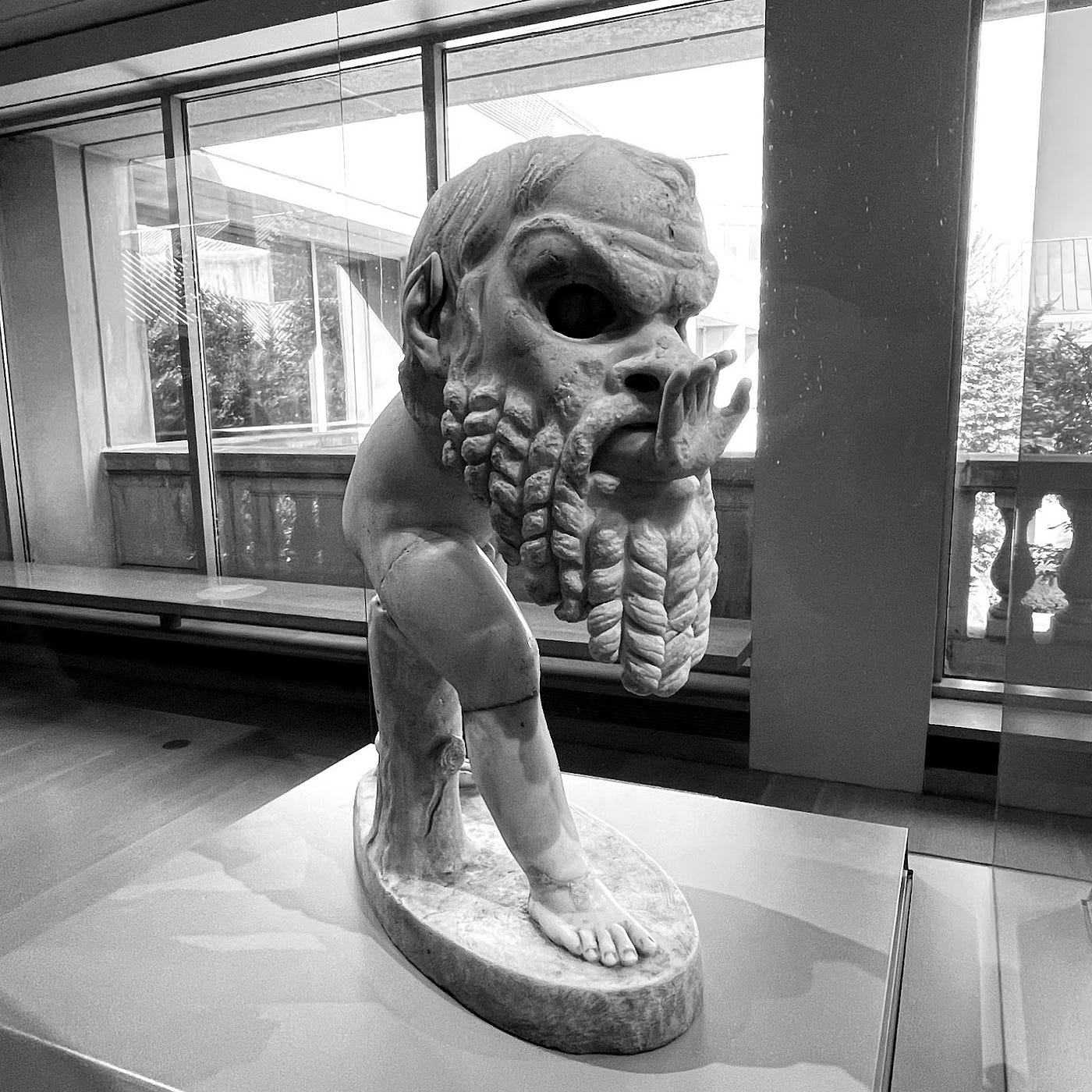This black and white photograph, likely taken during the daytime in a museum, captures an unusual and grotesque statue displayed on an elevated white platform with an oval base. The sculpture, situated indoors, shows a male figure with a disproportionately large head, adorned with carved hair and a visible right ear. Disturbingly, the head features large, hollow eye sockets and an open mouth from which a right hand extends outward, palm facing forward. The figure is missing its left leg, but the short, muscular right leg is visible, emerging from a stump beneath the figure's behind. The background reveals large windows through which daylight streams, and you can make out reflections of trees and possibly a walkway with a railing outside.